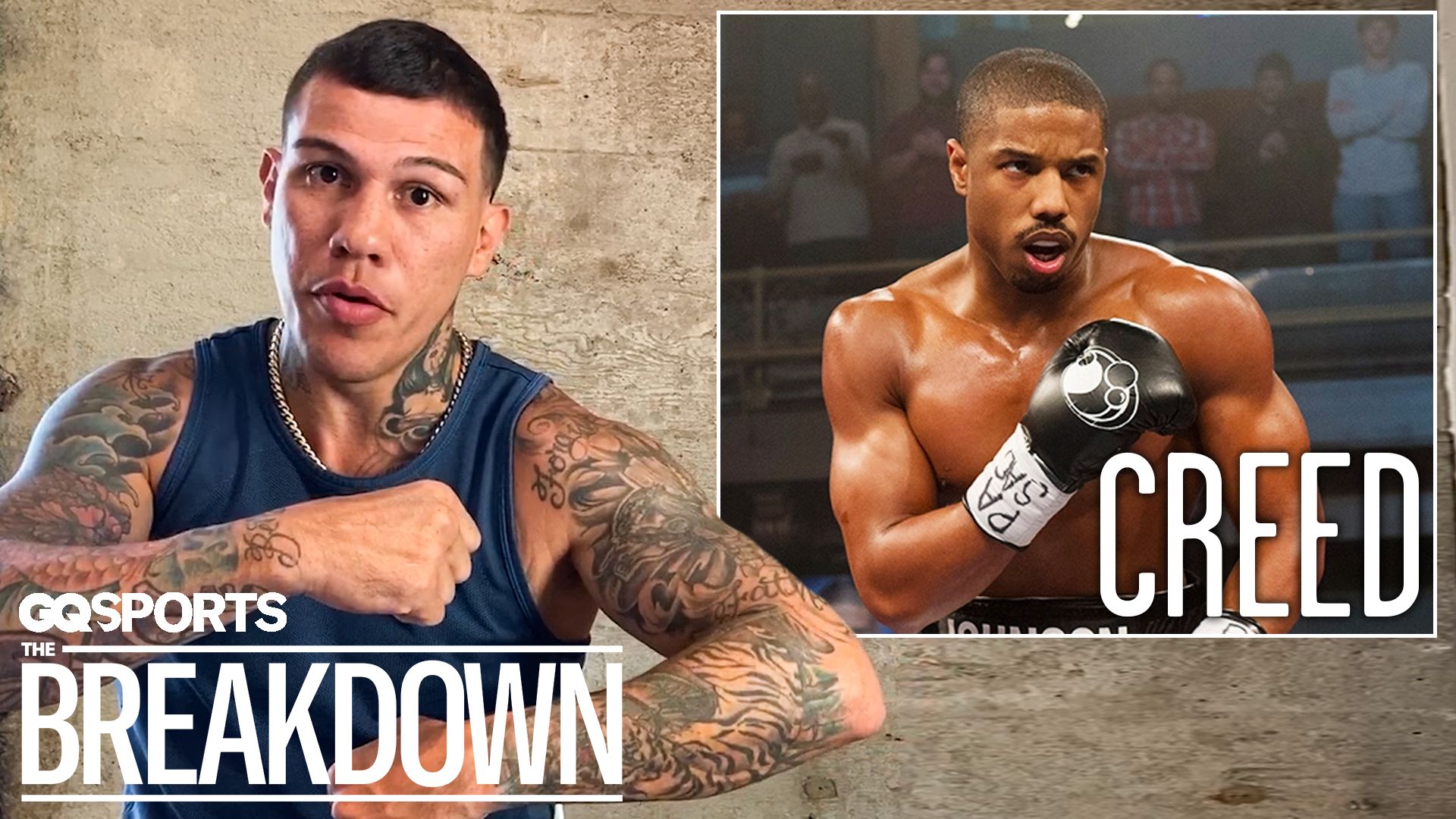The image is a color photograph featuring two figures positioned side-by-side, with a young Hispanic man prominently shown on the left. He is wearing a dark blue shirt and a gold chain, and his arms and neck are heavily tattooed. His pose mimics a defensive boxing stance, with his fists raised in front of his chest as though preparing to block or strike. In the lower-left corner of the image, white text reads "GQ Sports, The Breakdown."

On the right side of the image, there is an inlaid photo showing a shirtless, muscular African American man with a focused, intense expression. He is wearing black boxing gloves and is poised as if facing an opponent. The right corner of this smaller image features the word "Creed" in white letters, indicating a connection to the popular movie series.

The overall backdrop is a neutral, cement-like wall, and the layout suggests an advertisement or cover for GQ Sports, The Breakdown, possibly discussing the Creed movies or featuring an interview related to them. The Hispanic man's mimicking pose and the "Creed" lettering link the two images, emphasizing the boxing theme.